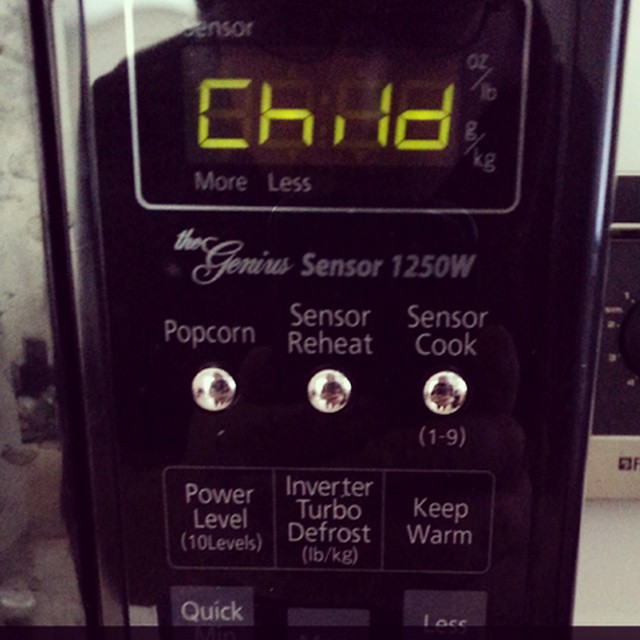This detailed color photograph captures a close-up view of the control panel of an old microwave oven. The microwave features a prominent digital display where the word "child" is oddly shown in yellow text at the top. Just below this, in smaller white text, it reads "sensor," and there are additional indicators for weight measurements: "ounce/pound" and "gram/kilogram." Centered on the panel is the phrase "The Genius Sensor, 1250 watts."

Below this central area, the control panel is described in greater detail. On the left, there are silver buttons for different cooking modes: "popcorn," "sensor reheat," and "sensor cook," with additional details such as "1-9" beneath "sensor cook." Further down, buttons labeled "power level" (with "10 levels" noted in parentheses), "inverter turbo defrost" (with "LB/kg" in parentheses), and "keep warm" are clearly visible. To the lower left, there is a button labeled "quick," and further to the right, another button labeled "less." The high reflectivity of the panel allows us to see the reflection of the person taking the photograph. The control panel is black with white and silver text, contributing to its classic appearance.